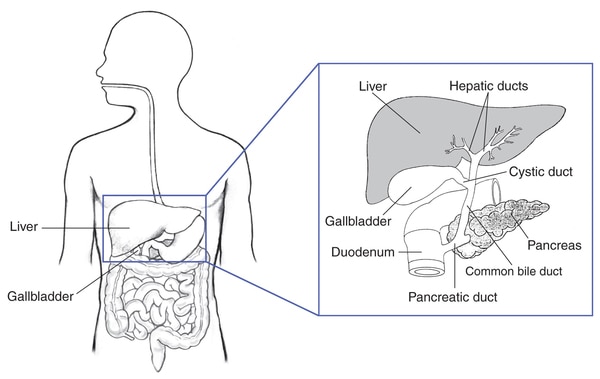The image is a detailed medical diagram depicting a male silhouette from the head down to just below the waistline, where the drawing ends. The silhouette is an outline, with the head turned sideways, and it shows the see-through internal organs. Key organs and parts of the digestive system are labeled, including the liver, hepatic ducts, cystic duct, pancreas, common bile duct, pancreatic duct, gallbladder, and duodenum. There is a focus on these organs, with lines pointing to the liver and its related ducts. Additionally, a zoomed-in square to the right provides a close-up view with detailed labels for these parts, clarifying their positions and interconnections within the body. This diagram serves as an educational tool to illustrate the liver's placement and its associated ducts in relation to other digestive system organs.